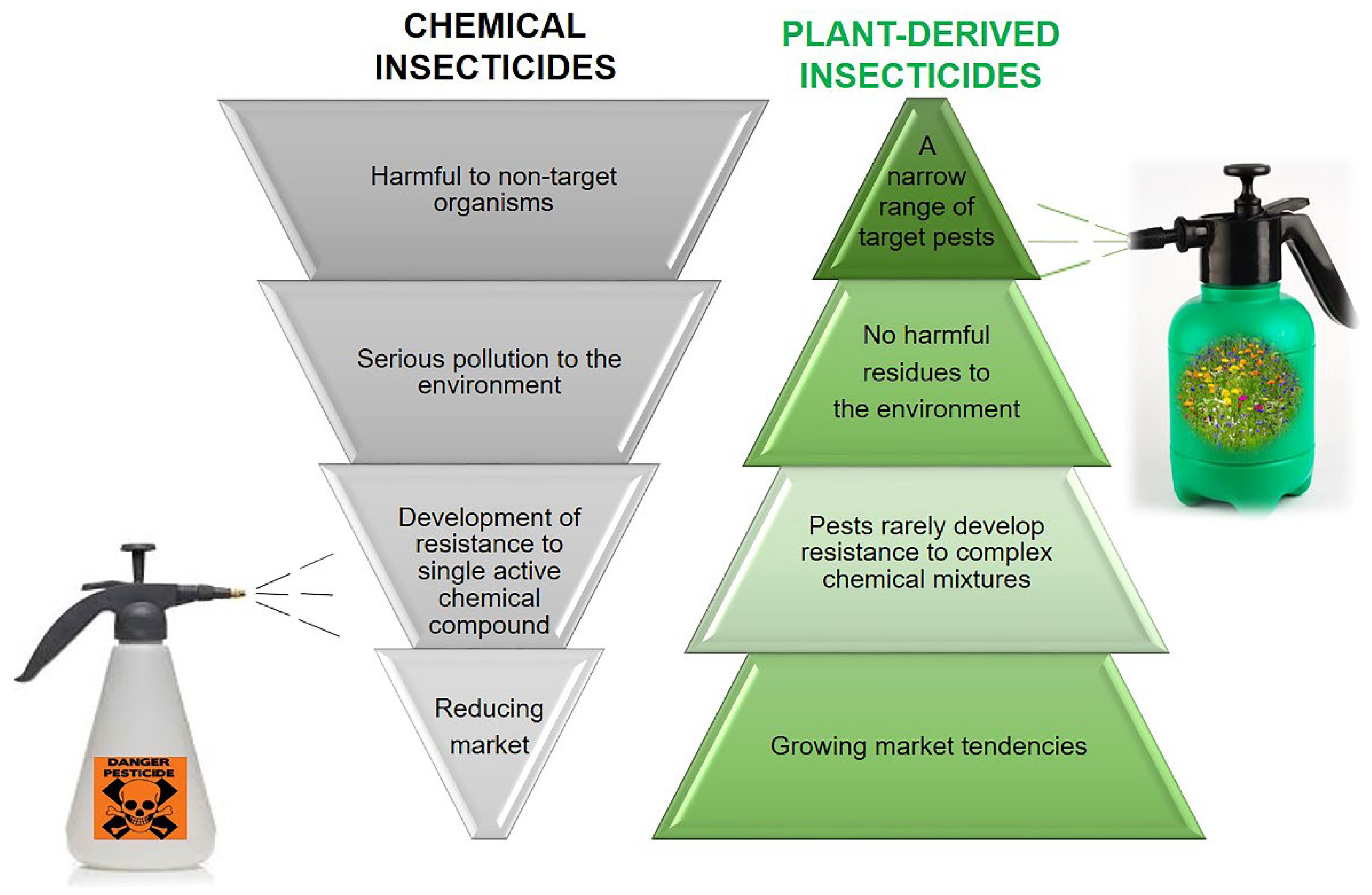The image is a detailed diagram comparing the impacts of chemical insecticides versus plant-derived insecticides, using two sets of color-coded triangles to illustrate the contrast. On the left side, gray overlapping downside-facing triangles represent chemical insecticides, topped with black text that reads "chemical insecticides." Each triangle contains a negative impact: "Harmful to non-target organisms," "Serious pollution to the environment," "Development of resistance to single active chemical compounds," and "Reducing market." Adjacent to these triangles is a white bottle labeled with a skull and crossbones, symbolizing danger, spraying its contents onto the gray triangles.

On the right side, a series of green upward-facing triangles signify plant-derived insecticides, with green text at the top that reads "plant-derived insecticides." Each triangle lists a positive attribute: "A narrow range of target pests," "No harmful residues to the environment," "Pests rarely develop resistance to complex chemical mixtures," and "Growing market tendencies." To the right of these triangles stands a green spray bottle with a black nozzle, also depicted as spraying its contents onto the green triangles, giving an inviting appearance with a more eco-friendly and beneficial depiction. The visual contrast clearly highlights the negatives of chemical insecticides against the positives of plant-derived alternatives.